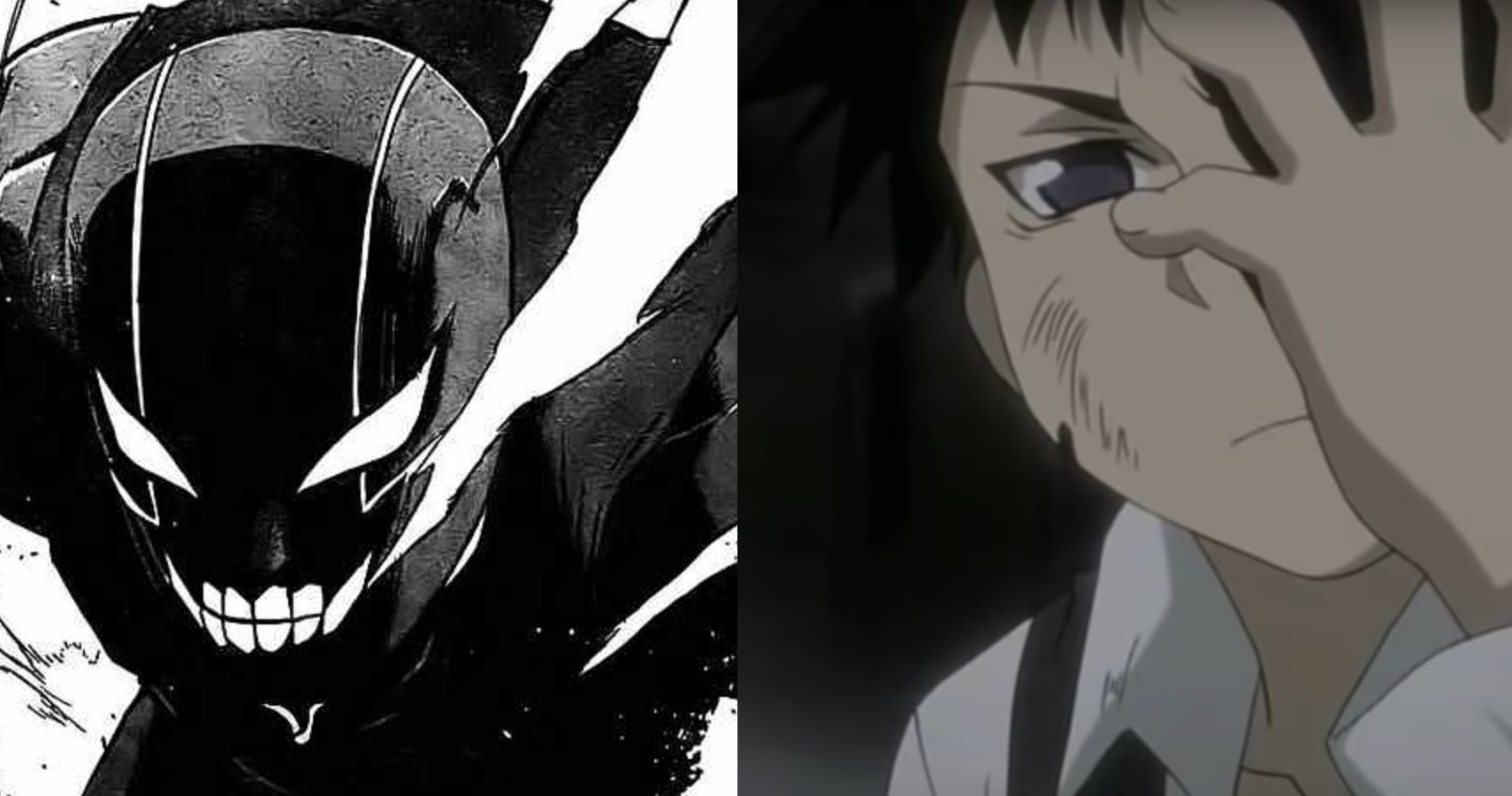The landscape-oriented image is a combination of two distinct, hand-drawn illustrations set side-by-side, both square in format. On the left, the haunting black-and-white illustration features a demonic figure with an eerie, alien-like appearance. Characterized by its big, pointy eyes reminiscent of an alien, the figure's black mask has white slits for eyes and a sinister mouth that resembles skeleton teeth. Two white streaks trail down from the top of its head, giving a sense of rapid movement. This menacing figure is captured from the head to below the chin, exuding an overall evil aura. 

On the right, a detailed, color anime-style drawing portrays a worried young male with spiky black hair, a big gray eye, and light tan skin. He is depicted from the forehead to the neck, with his hand covering his left eye, leaving only his right eye visible. Donned in a white collared shirt, the boy is set against a black background, conveying a sense of unease and introspection. The juxtaposition of the two images creates a striking contrast between the demonic and the human, each rendered in their respective stylistic nuances.